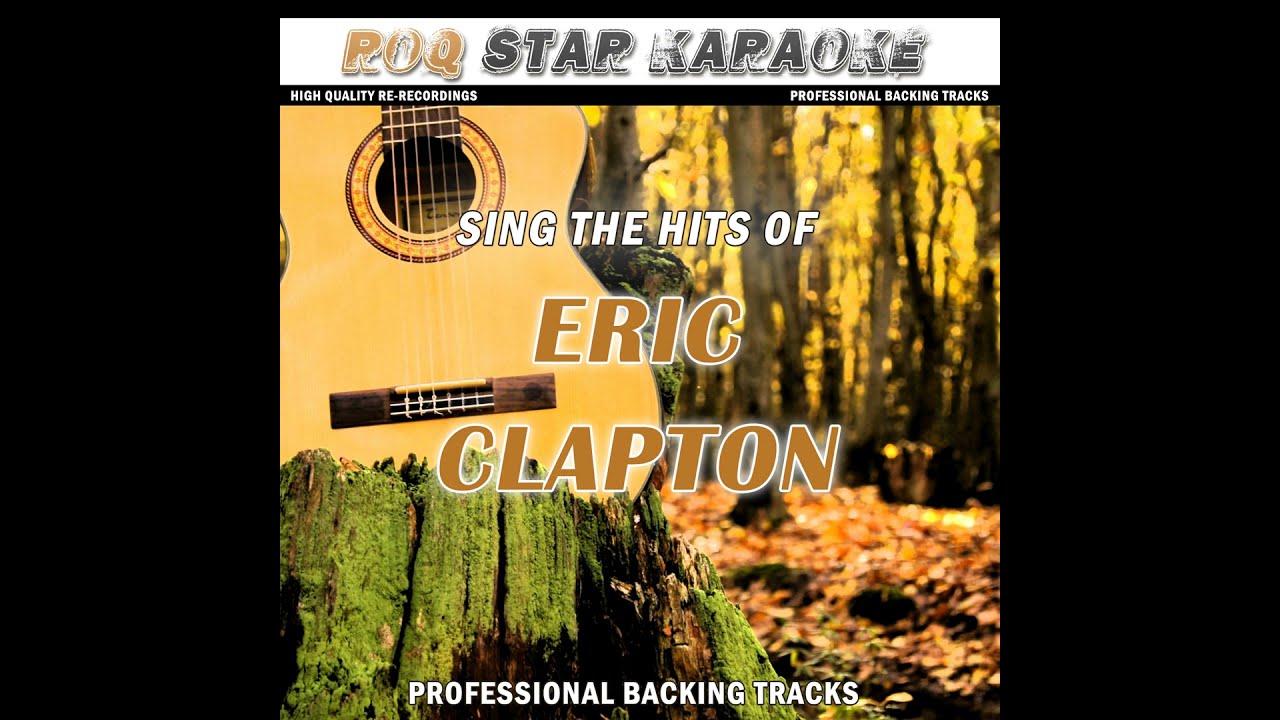The image depicts a promotional cover for R.O.Q Star Karaoke. Dominating the scene is a detailed guitar placed prominently in a forest setting. The guitar, shown from the top and featuring six strings, rests against a moss-covered tree stump surrounded by lush foliage and bare trees. Overlaid text in bold, brown, and blocky fonts announces "Sing the Hits of Eric Clapton," emphasizing the karaoke focus. At the top of the image, "R.O.Q Star Karaoke" is displayed within the header, featuring some intricate and flashy graphical elements. Below this header, a thin black band states on the left "High Quality Re-Recordings" and on the right "Professional Backing Tracks." The entire scene evokes a tranquil yet inviting environment that contrasts the earthy natural background with the musical promotion of Eric Clapton's hits.